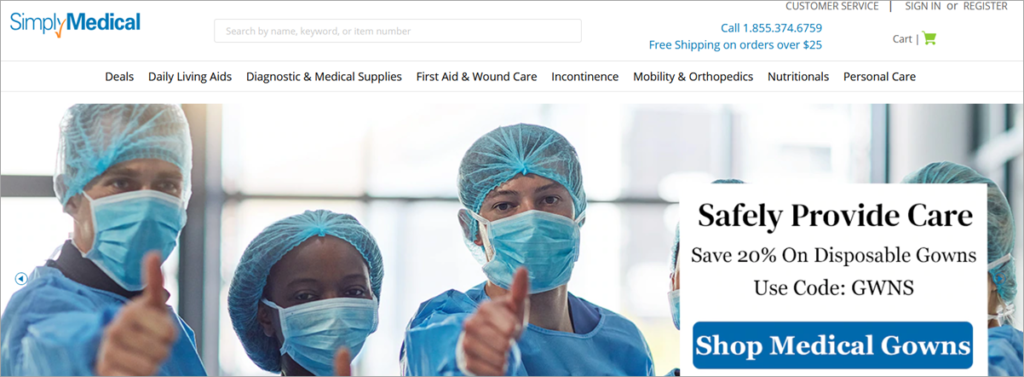Screenshot of Simply Medical Website

The image is a color screenshot of the upper portion of the Simply Medical website. At the top, "Simply Medical" is prominently displayed in blue text, separated by an orange checkmark. Below the logo is a search bar, allowing users to search by name, keyword, or item number. 

In the top right corner, there are options to access customer service, sign in or register, and a direct call button with the customer service number 1-855-374-6759 (US country code: 001). The website also advertises free shipping on orders over $25, emphasizing its role as a shopping site for medical equipment.

A cart icon is visible, indicating no current items inside since there is no number next to it. The navigation bar features various categories including Deals, Daily Living Aids, Diagnostic and Medical Supplies, First Aid and Wound Care, Incontinence, Mobility and Orthopedics, Nutritionals, and Personal Care.

A promotional banner announces a 20% discount on disposable gowns with the code 'GWNS'. An image accompanying the promotion shows a group of surgeons or doctors giving thumbs up, engaging directly with the viewer.